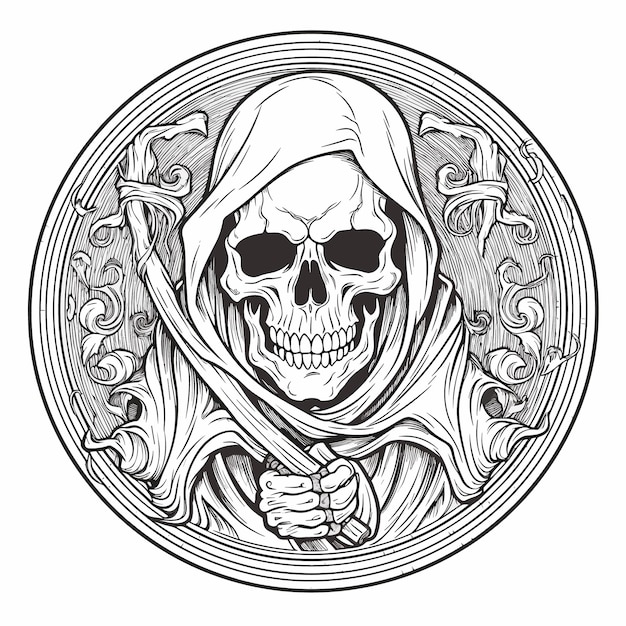The illustration depicts a skeletal figure, reminiscent of the Grim Reaper, centered within a circular design. The skeleton, facing directly towards the viewer, is adorned with a white hood and draped in tattered white fabric, which appears to float upwards like wisps of smoke. It holds a staff-like object, possibly made of bones, that curves slightly to the right near the top. The figure's hands are positioned just below its skull, which features dark eye sockets and nasal cavities, enhancing its eerie appearance.

Surrounding the skeleton is a series of concentric circles, creating a spiral effect with dark grey shadings that intensify towards the center. Floral designs embellish either side of the skeleton, adding a contrasting delicate touch to the macabre scene. The entire circular motif is bordered by a thick black line, set against a stark white background. The dark and ghostly aesthetic of the image is accentuated by the detailed shadings and the floating, ethereal quality of the fabric.